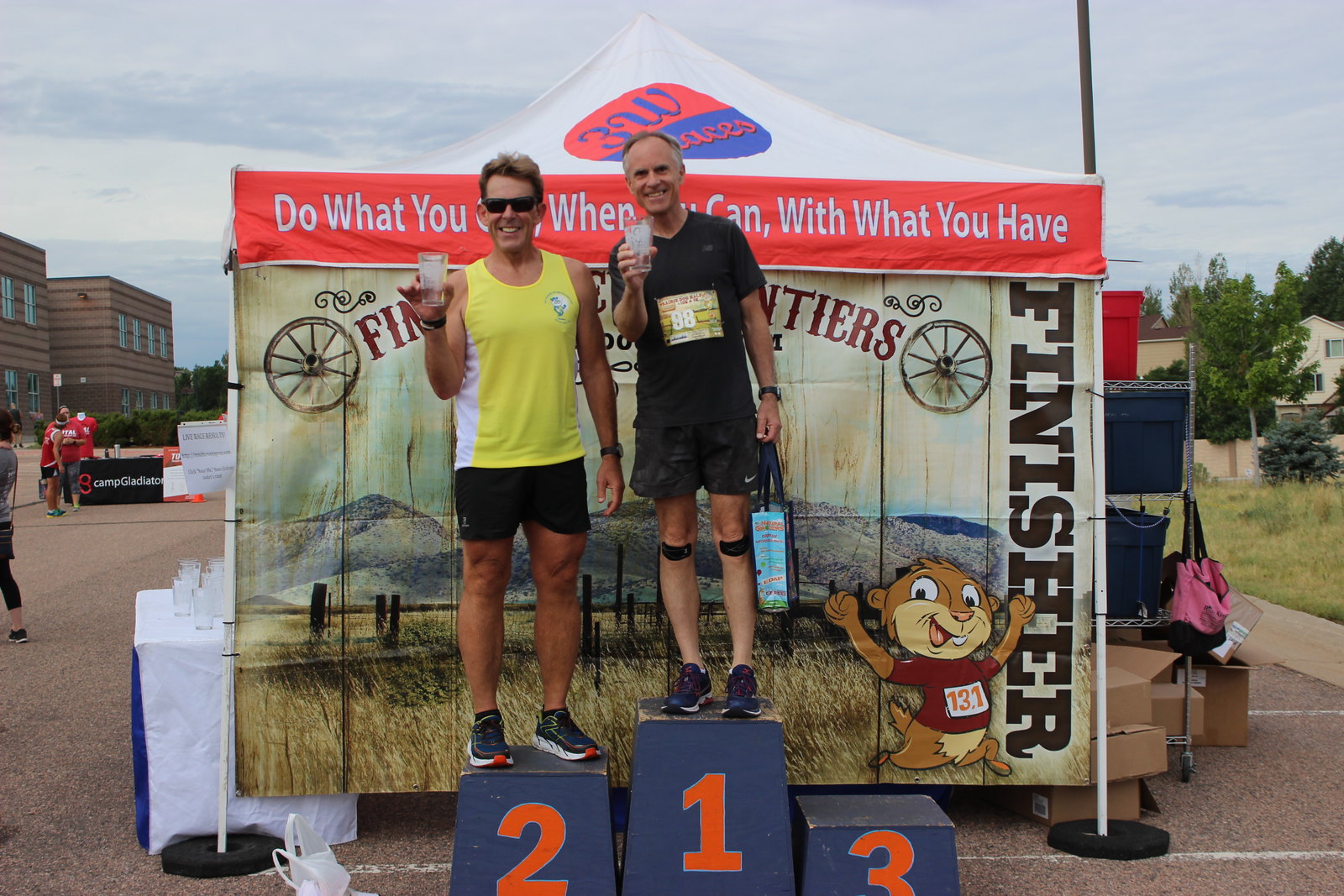In this detailed, full-color photograph taken outdoors on an overcast day, two men stand proudly on runners' blocks, each adorned with large orange numbers. The runners' block, positioned in the center of the image, consists of three different-sized square stands. The tallest stand, number 1, is on the far right, and it features a man wearing a black V-neck graphic short-sleeve t-shirt and black shorts. He sports two black Band-Aids on his knees and blue shoes, and he holds a blue tote bag with black handles. His graying hair suggests he is older, and he smiles directly at the camera. 

To the left, on the second-tallest stand with the number 2, stands another man who is early middle-aged, wearing a sleeveless yellow shirt with white stripes down the sides, black shorts, black shoes with white soles, and black sunglasses. He, too, smiles warmly at the camera. 

The shortest stand, numbered 3, remains unoccupied. In the background, a sign reading, "Do what you do when you can with what you have," is visible. Trees, a yellow two-story house, a table with a logo, and a brown two-story building can be seen as well. Below the sign, rolling hills, a western grassy field with a wooden fence, and a cartoon rodent creature wearing the number 13.1 add to the picturesque setting. The overall scene suggests a celebratory moment following some type of event or race.